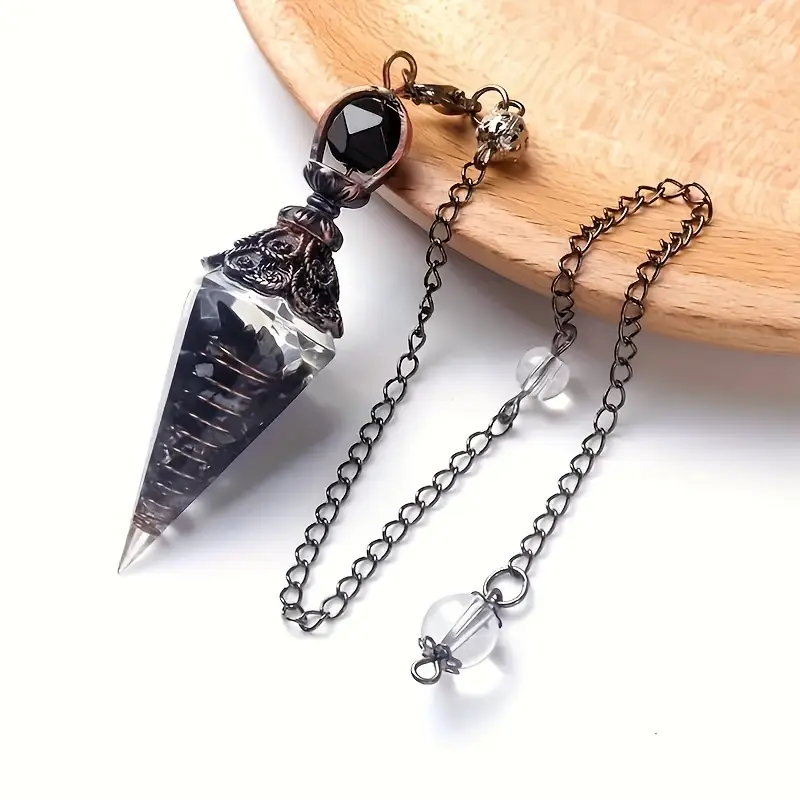This color photograph showcases a striking piece of jewelry set against a stark white background, occupying the left and bottom two-thirds of the image. The top right one-third features a shallow, light-colored wooden bowl, upon which the pendant rests. The pendant itself is a long, conical piece of glass with black tints, encasing a spiral of wire. At the top of the pendant, a silver inlay forms a horseshoe pattern, leading up to intricate decorations and a U-shaped piece that connects to a chain. Within this U-shaped segment lies a faceted black glass gem. A silver chain, comprised of tightly knit dark metal links, extends from the pendant. The chain loops down, back up, and over the wooden bowl, adorned with a clear glass bead halfway along its length and terminating in another clear glass bead. At the very top of the chain, a small silver bead is visible. The overall composition of the image emphasizes the sharp, pendulum-like shape of the pendant, with its clear glass tip and dark, intricate metalwork detailing.